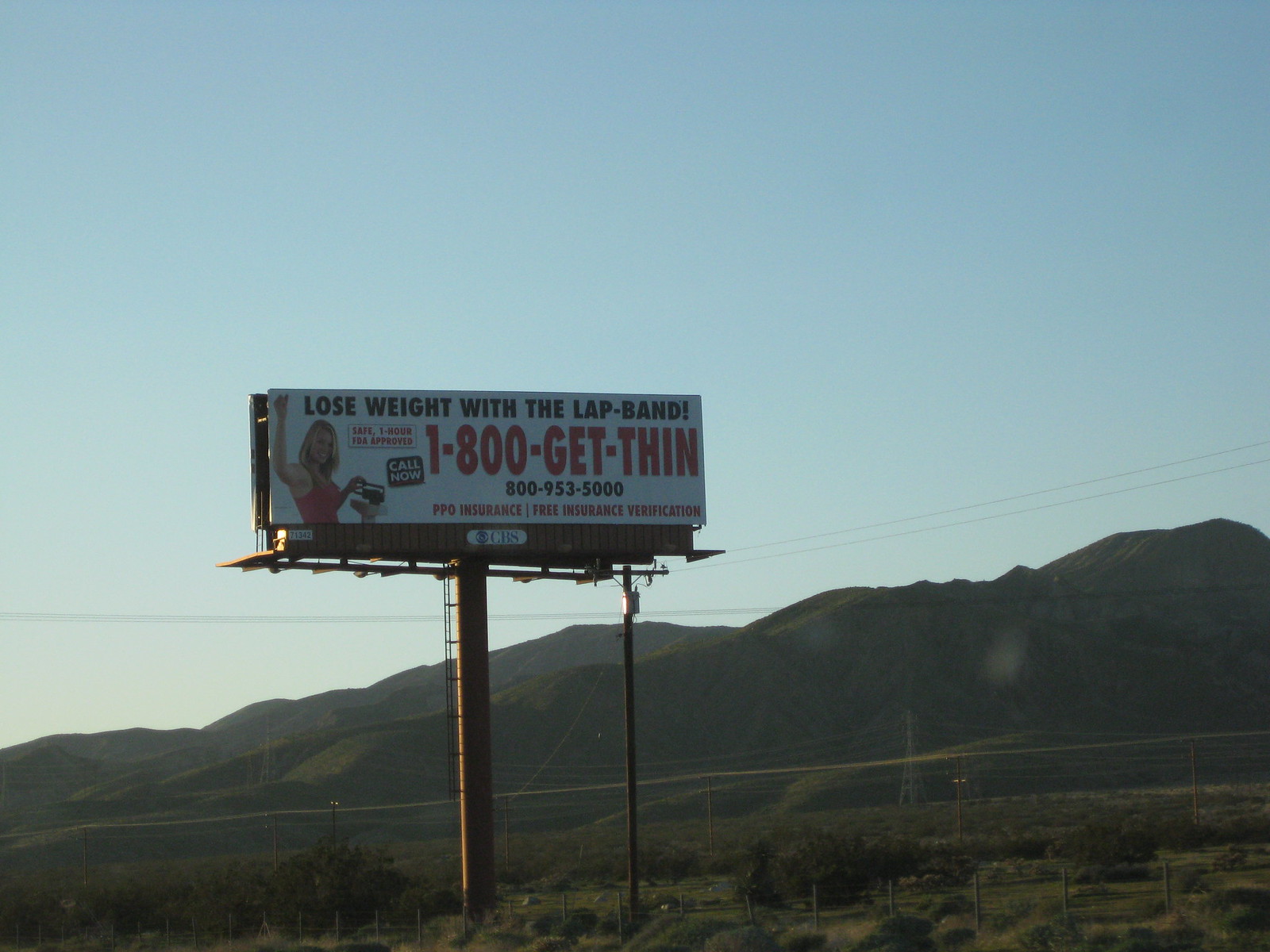In this outdoor photograph, the distant landscape features verdant, rolling mountains or tall hills, likely covered with dense greenery, including trees and grass. The scene is set against a backdrop of a clear, pale blue sky, giving the image a serene atmosphere. In the foreground, there is an open field dotted with various shrubs and small plants, enclosed by a wooden fence. Dominating the lower portion of the image is a large billboard supported by a sturdy structure. The billboard prominently advertises a weight loss method with the slogan "Lose weight with the Lap-Band," accompanied by the phone number 1-800-GET-THIN. The billboard is designed with a white background and features a picture of a smiling blonde woman wearing a red tank top, her hand resting on a bathroom scale, presumably illustrating the success of the advertised weight loss method.